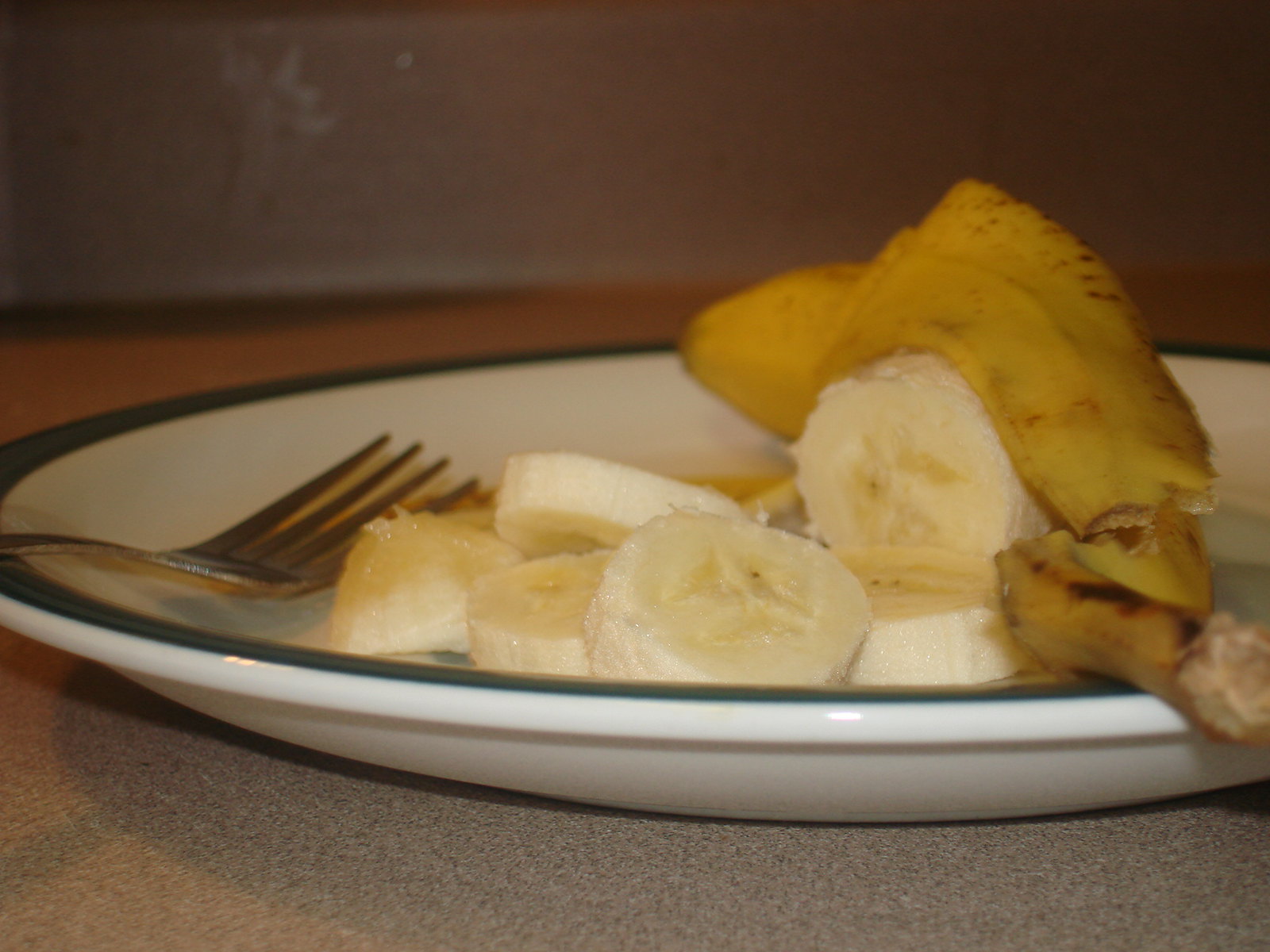In the image, set against a dark background with hints of brown on the floor, there is a gray, heavily spotted countertop featuring numerous black spots. At the center of the composition, a white dish is prominently displayed, casting subtle shadows underneath. On the left-hand side of the dish rests a silver fork. The rim of the dish is distinctly marked with black accents.

Positioned in the middle of the dish is a neat pile of six banana slices. Draped over these slices is the banana peel, extending from front to back. The yellow peel, adorned with brown spots, reveals a portion where it has cracked or cut away from the stem, showing a brownish area indicative of the point of detachment. The banana slices themselves appear moist, suggesting ripeness with some pieces displaying the characteristic wetness that indicates natural sweetness due to sugar conversion.

The scene is illuminated solely by the flash of the camera, accentuating the textures and details of both the banana slices and the speckled countertop.